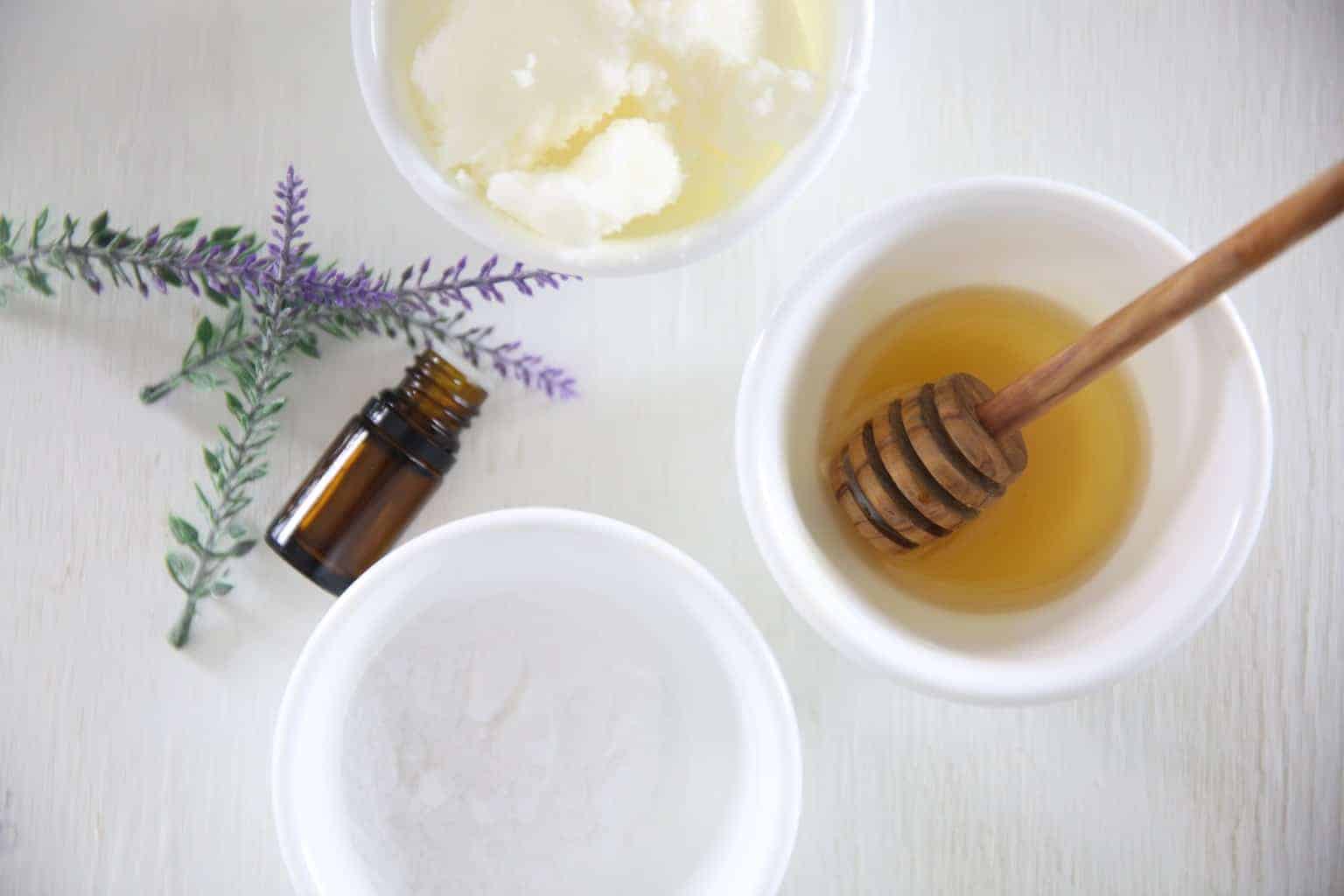In this overhead scene, we see three white bowls arranged on a white surface. The bottom-left bowl appears either empty or holds water, with shadows making it difficult to distinguish. In the middle, right side, there's a bowl containing a viscous, amber-colored substance, likely honey, accompanied by a long-handled wooden honey dipper with circular cutouts. The top-left bowl contains a mysterious white substance, with its exact nature indeterminate. On the left side, there are sprigs of lavender wildflowers with green leaves transitioning to purple at the tips, lying atop one another. Beside these flowers is a small brown glass vial. This serene arrangement highlights a minimalist aesthetic, blending culinary and natural elements.